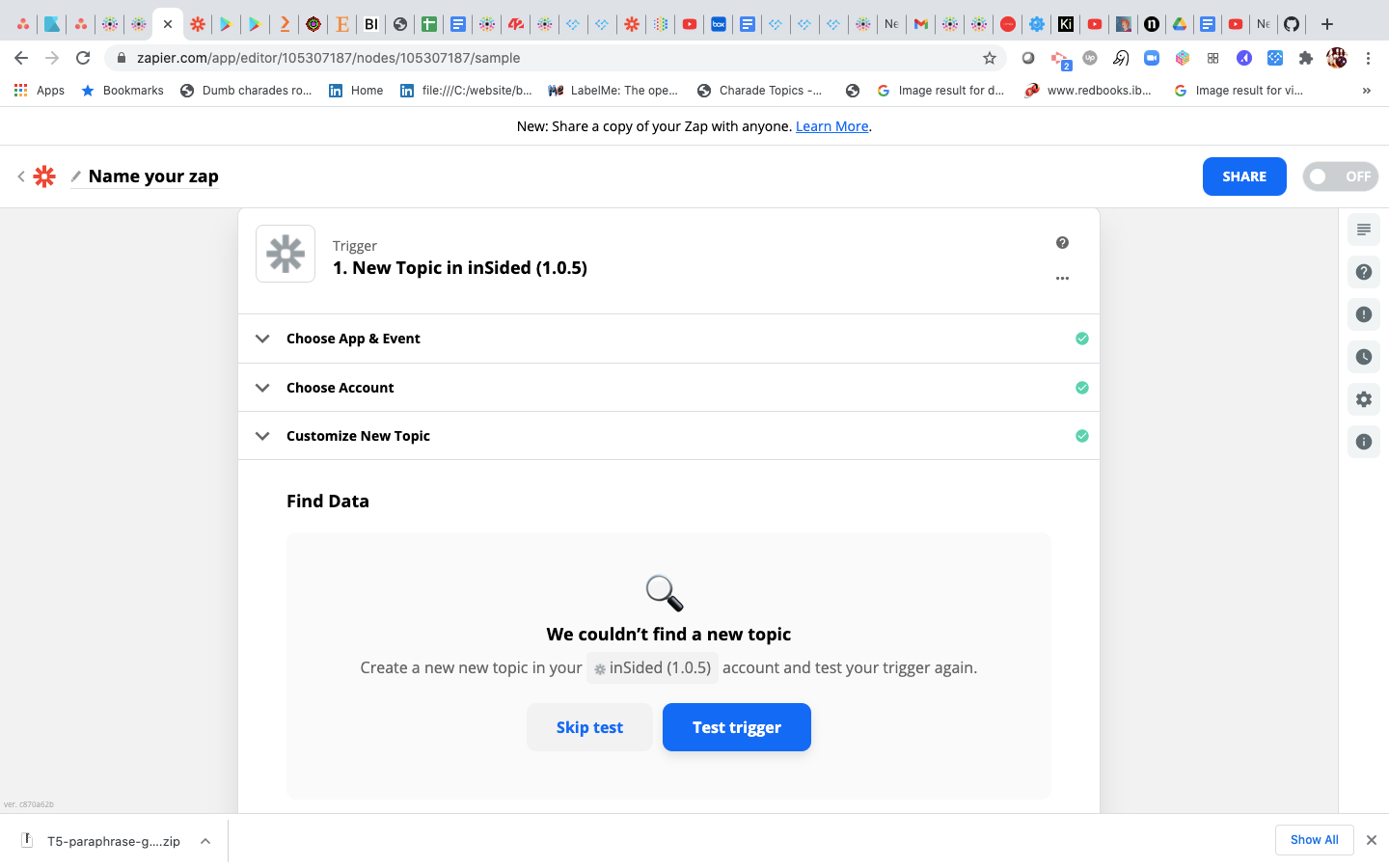In this screenshot, we see a Chrome browser window open with numerous tabs so minimized that only the website icons are visible. The URL in the address bar indicates the user is on zapier.com. At the top of the webpage, there's a header that reads, "New: Share a copy of your Zap with anyone," followed by a "learn more" link in blue text. Directly beneath, a flower-like logo represents Zapier.

The page prompts the user to "Name your Zap." To the right of this, there's a blue "Share" button and a toggle switch to activate or deactivate the Zap. Moving further down, there's a grey flower logo alongside the word "Trigger," followed by the text, "One new topic in Insighted (1.0.5)," all in black font.

Subsequently, the section is divided into outlined steps: "Choose App and Event," "Choose Account," and "Customize New Topic." Each of these sections includes drop-down arrows indicating the availability of further options. At the bottom of the screen, the message, "Find Data," displays the result, which indicates no new topics were found with the prompt, "Create a new topic in your Insighted account and test your trigger again."

This area also features two buttons: "Skip Test" in blue font within a grey box on the left, and a blue "Test Trigger" button with white text on the right.